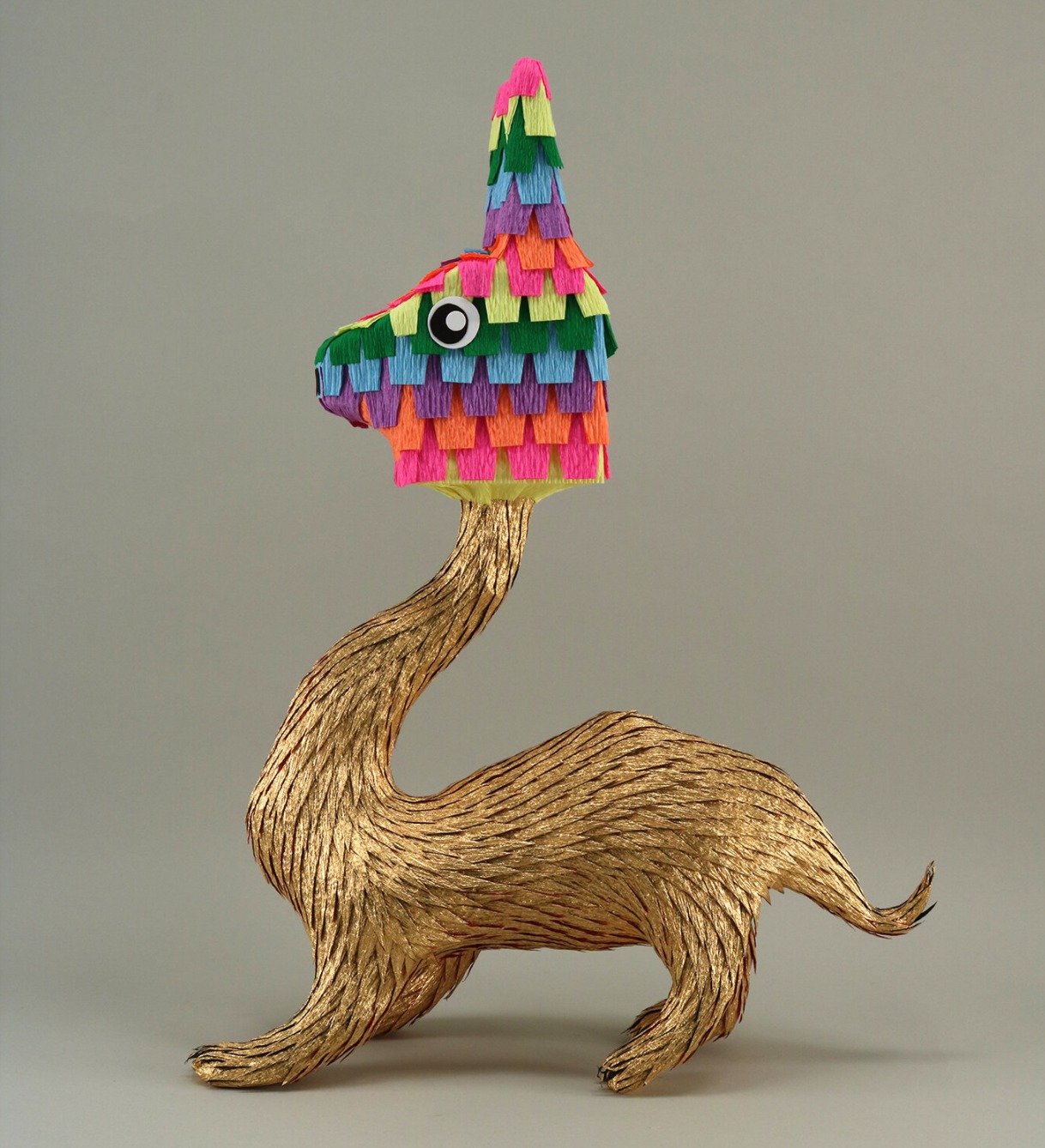This professional photograph captures a whimsical, three-dimensional piece of artwork that combines elements of various animals. The creature features a small mammal-like body and a long, upward-curving neck, reminiscent of a cat or weasel, but it sports the head of a llama or alpaca designed with colorful, pinata-like materials. The head is adorned with overlapping pieces of vibrant fabric in shades of pink, yellow, green, blue, purple, and orange, and it has a googly eye composed of concentric circles in white and black.

The body of the creature appears to be crafted from a bronze-like metal, giving the impression of fur with its textured surface. It stands on four legs, has a slightly curled tail, and is placed on a professional photo mat. The background and floor are a dark beige or gray, adding contrast that highlights the colorful and imaginative nature of the artwork. The overall feel of this piece is one of whimsy and playfulness, capturing attention with its unconventional and creative design.